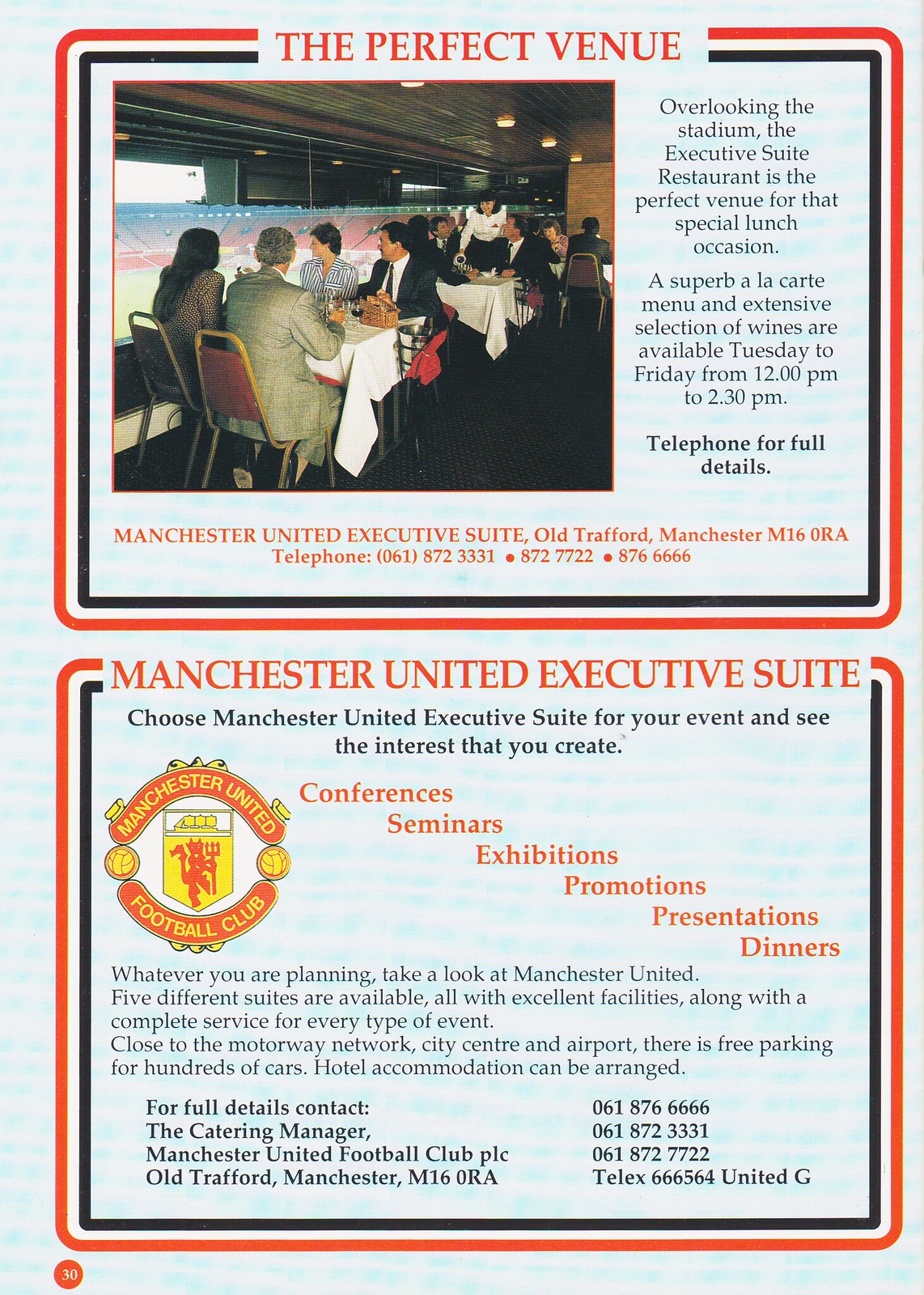This tall rectangular advertisement, featuring a light bluish-white background, is promoting the Manchester United Executive Suites at Old Trafford, emphasizing its suitability for various events. The page is structured into two sections, each bordered by a series of red, white, and black curving lines. At the top, the caption reads in bold red font, "The Perfect Venue." Beneath this, there's a photograph depicting several people dining in a luxurious skybox-style restaurant with a clear view of the stadium field below.

The accompanying text praises the Executive Suite Restaurant for its superb à la carte menu and extensive wine selection, available Tuesday to Friday from 12 PM to 2:30 PM. It highlights the venue as ideal for special lunch occasions. Contact information includes multiple phone numbers: 061-872 3331, 872 7722, and 876 6666. 

The advertisement also promotes the Manchester United Executive Suites for events such as conferences, seminars, exhibitions, promotions, presentations, and dinners, stating, "Choose Manchester United Executive Suites for your event and see the interest that you create." It mentions that there are five different suites available, all equipped with excellent facilities and complete service for any event type. The location is noted for its proximity to the motorway network, city center, and airport, and it provides free parking for hundreds of cars with hotel accommodation available upon request. The crest of Manchester United is also featured prominently in the design, reinforcing the brand's identity. Predominant colors in the advertisement are black, red, and white, maintaining a professional and visually appealing aesthetic.